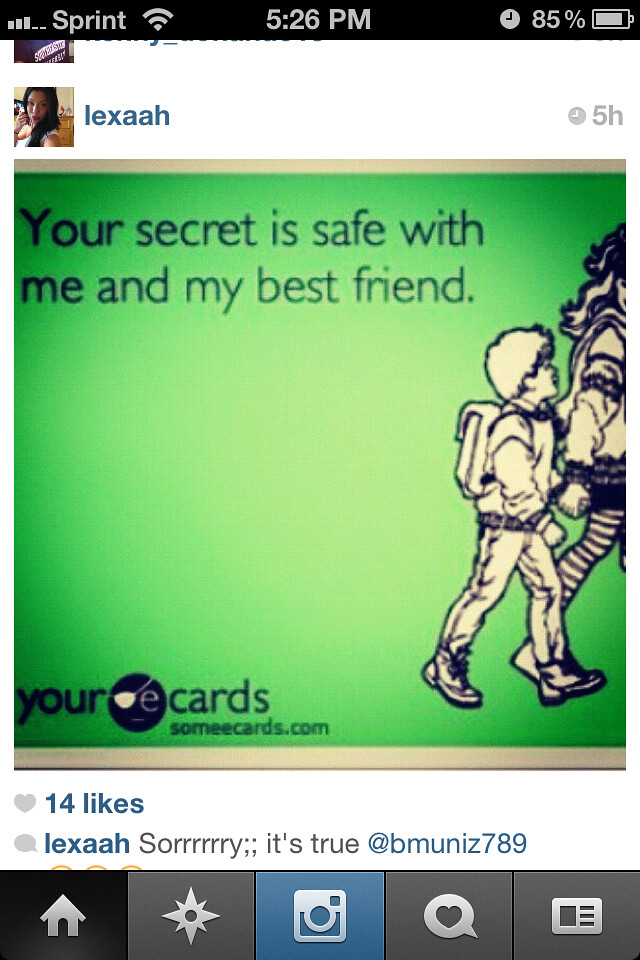The image is a screen grab of an Instagram post, taken from a smartphone. At the very top of the screen, on a black bar, are various elements of the phone’s UI, including a weak cell signal, the word "Sprint" in white text, the time displayed as 5:26 PM, a clock symbol indicating an alarm set, an 85% battery percentage, and a fully charged battery icon. At the bottom of the screen are five navigation buttons: a stylized white house, a compass, a blue and white camera, a speech bubble with a heart inside, and a rectangle with four smaller rectangles within it.

The Instagram post itself features an e-card with a green background. The text on the card reads, "Your secret is safe with me and my best friend." The card includes a black-and-white illustration partially cropped on the left and right sides. The illustration depicts a girl, mostly cropped out, with long hair, wearing a white jacket, a black skirt, and black and white striped thigh-high socks. The girl is holding the hand of a younger boy with a backpack, blue jeans, and tennis shoes, who is looking up at her.

The top-left corner of the Instagram post shows a square avatar of a white woman with black hair, next to the username "Lexaah" in blue text on a white background, followed by "5H" indicating the post was made five hours ago. In the bottom-left corner of the e-card is the logo "your e-cards," with the "E" inside a black circle featuring an eyepatch. Below that is "someecards.com." The post has 14 likes, and Lexaah comments, "sorry it's true," tagging @Bmunids789. The Instagram navigation buttons are dark brown, with icons including home, explore (a star), a camera, a text bubble with a heart, and a square with horizontal lines.